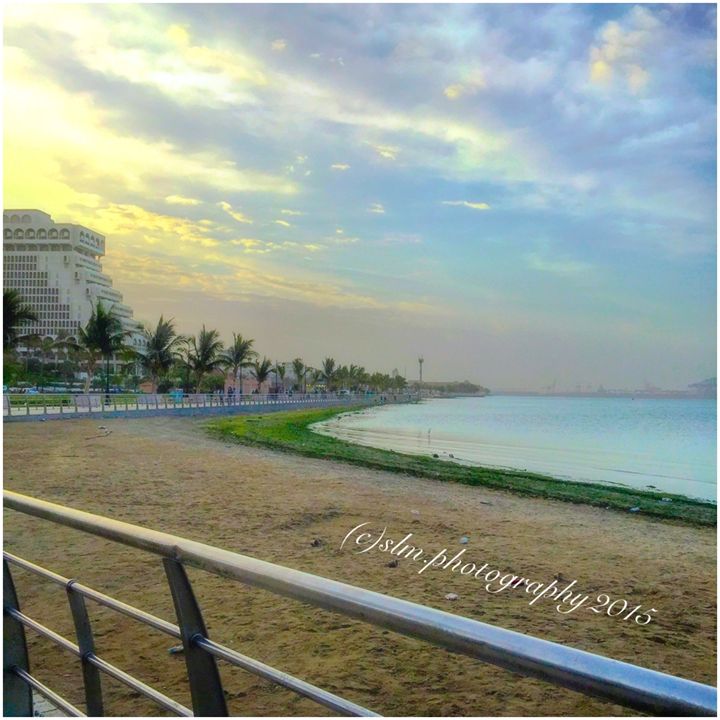This square photograph, resembling a postcard, captures a serene beachfront scene likely from a developed resort area, possibly in Florida. The image is taken from behind a silver railing or fence that traverses diagonally across the bottom half, forming a barrier along a boardwalk. In the foreground, the yellow-tinted sandy beach, marked by numerous footprints, meets a green patch of grass that lines the calm, light blue water, suggesting a bay with minimal waves.

Above, the sky transitions from a clear blue at the top to a vibrant yellow near the horizon, indicative of either dawn or dusk. Wispy, partially cloudy skies with hues of light purple and peach are illuminated by the sun, which sits off to the left side.

The background features numerous palm trees lining a road, creating a picturesque tropical atmosphere. Dominating the scene is a large, white terraced hotel with a grid of numerous square windows, reminiscent of a pyramid shape with cascading stories. Additional structures, possibly other hotels or restaurants, are scattered throughout, reinforcing the impression of a busy resort locale. 

A copyright notice in white text reads "SLM.photography 2015," confirming the work of a professional photographer.